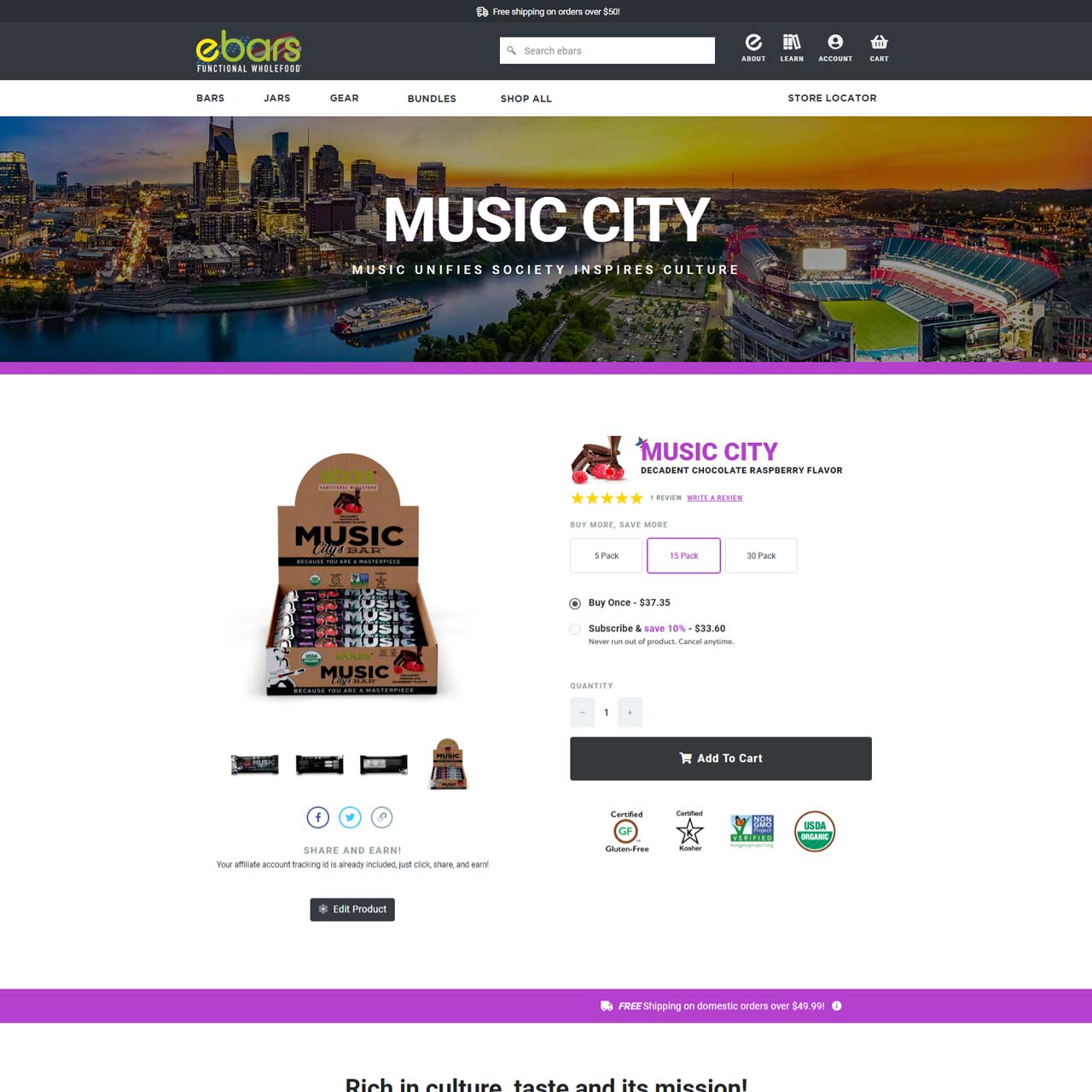This screenshot showcases the "Music City Chocolate" product page on the eBars website, known for its functional whole foods. At the top left corner, "Functional Whole Foods" is prominently displayed. The top navigation bar includes a truck icon accompanied by "Free shipping on orders over $50." Below that, a search bar labeled "Search eBars" is centered, flanked by navigation links for About, Learn, Account, and Cart on the right.

The secondary navigation bar offers links to Bars, Jars, Gear, Bundle, Shop All, and a Store Locator on the far right.

The main content area is dedicated to the "Music City" product, subtitled "Music unifies society, inspires culture." A city skyline and a stadium serve as the page's backdrop. The highlight of this page is the Music City Chocolate product, featuring a decadent chocolate raspberry flavor. A mouth-watering image shows raspberries being coated in rich chocolate.

The product boasts a perfect five-star rating from one review, with a purple link inviting customers to write a review. There's a "Buy More, Save More" promotion, allowing customers to choose between a 5-pack, 15-pack (highlighted), and a 30-pack. Pricing options are given for one-time purchases at $37.35 or a subscription plan offering a 10% discount for $33.60, with the benefit of never running out and the flexibility to cancel at any time.

An appealing image of all the product bars neatly packed in a box is displayed. On the left, there's an option to "Share and Earn." Certification labels including Certified Gluten-Free, Certified Culture, Non-GMO, and USDA Organic are prominently featured to assure quality and authenticity.

At the bottom, a banner reiterates "Free shipping on domestic orders over $49.99," rounding off this detailed and enticing product page.